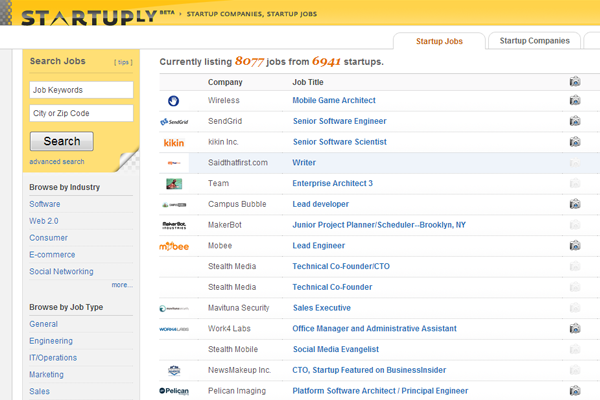In this image, we see a horizontally-oriented screenshot of a web page. The top portion of the screen is highlighted in a bright yellow color featuring the company's name in bold black text, accompanied by the word "Beta" in smaller text to the right. Directly below this, against a white background, we see two navigational tabs: one labeled "Start Up Jobs" in dark gray text, which is currently active, and another labeled "Start Up Companies" in blue text to its right.

Further down, in blue text, the web page indicates that there are currently 8,077 jobs from 6,941 startups listed. This announcement is accentuated with the job count in red text. Following this, the content is structured into two columns, one for the company name and the other for the job title.

The first entry lists the company "Wireless" with the job title "Mobile Game Architect" in blue text. The second entry shows the company "SendGrid" and the job title "Senior Software Engineer" in blue text. The third entry features "Kickin, Inc." and the position "Senior Software Scientist."

The layout is clean and organized, primarily using a text-based approach to display the job opportunities available across various startup companies.